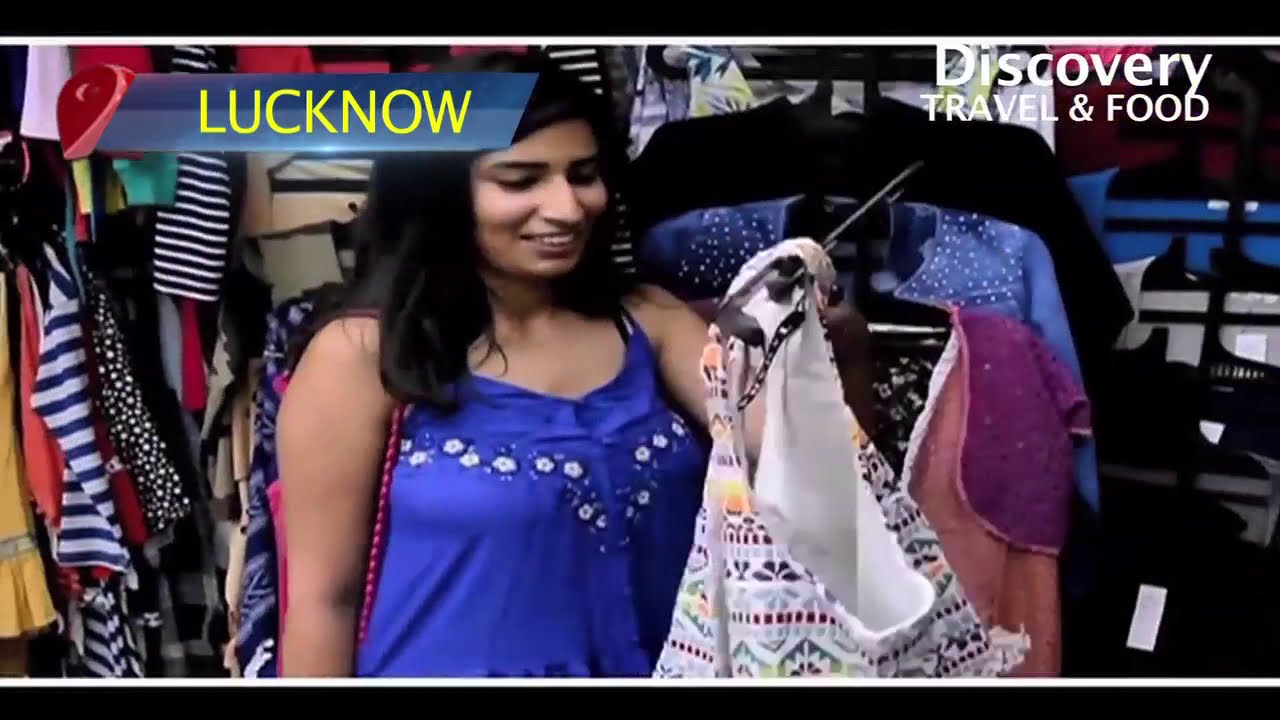In a clothing store filled with vibrant garments in shades of blue, white, purple, pink, black, brown, red, yellow, and gray, a woman with long black hair, possibly Indian and with darker skin, stands slightly off-center to the left. She is dressed in a sleeveless blue top adorned with a floral pattern along the bosom and down the center. With a smile on her face, she holds up a white tank top on a hanger. The scene is well-lit, highlighting the arrays of clothes on racks and hangers behind her. This image looks like a screenshot from a TV show or YouTube video, reinforced by graphical text elements. In the upper left corner, within a semi-transparent blue parallelogram, the text reads "Luck Now." In the upper right corner, white text spells out "Discovery Travel and Food."